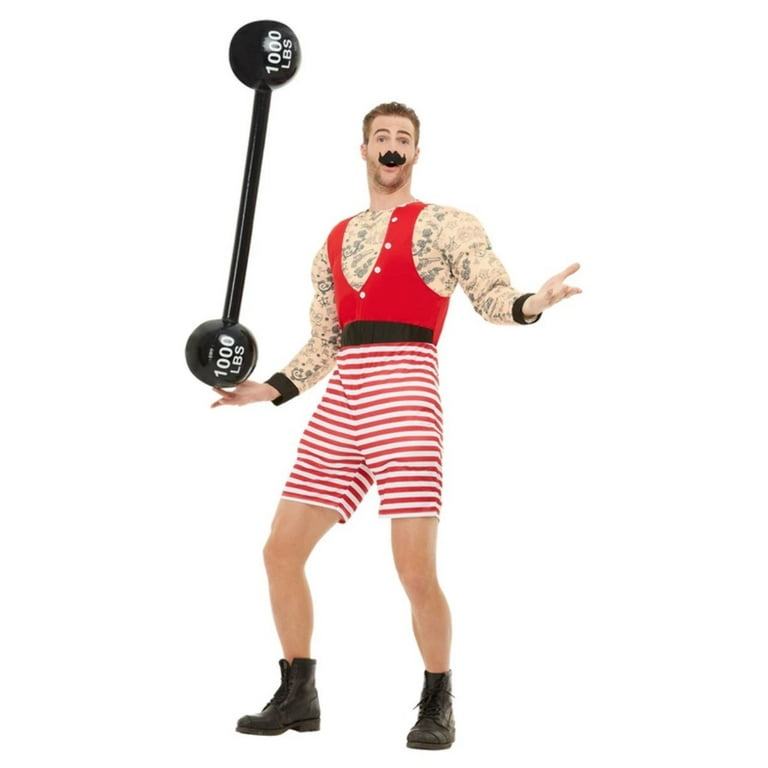The image portrays a man standing against a blank white background, resembling a product image often seen on Amazon or other listing pages. The man is styled to look like an old-timey strongman from carnival shows. He has short brown hair and a small beard, along with a notably fake, cartoonish black mustache. He wears a bright red vest over an intricately designed black and white shirt with paisley patterns and black collars on the wrists. His lower half is clad in red and white striped shorts that end just above his knees, complemented by black work boots. 

In his right hand, held effortlessly between his thumb and forefinger, is a black barbell with round ends labeled "1,000 pounds" in white letters, suggesting it is a gag or a prop for a magic trick. His left arm is raised with his palm up, adding to the whimsical pose. The man's outfit and expression suggest he could be dressed for a masquerade party or similar festive occasion, blending humor with an old-fashioned strongman aesthetic.